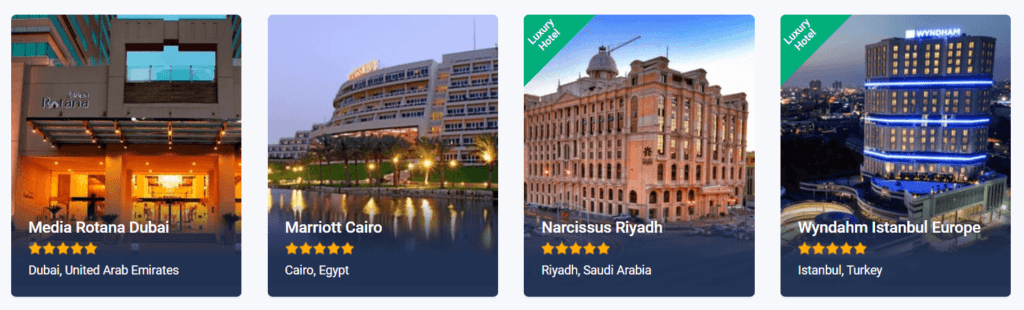The page features a collection of four high-quality photographs of various hotels from around the world, arranged sequentially from left to right across the page. 

1. **Media Rotana Dubai, Dubai, United Arab Emirates**: The first image captures the illuminated exterior of the Media Rotana Dubai, a prestigious five-star hotel. The bottom floor is brightly lit, showcasing the hotel's entrance. Above the entrance, the hotel's name is prominently displayed in elegant letters, along with five yellow-filled stars, indicating its luxury status. The caption underneath confirms its location as Dubai, United Arab Emirates.

2. **Marriott Cairo, Cairo, Egypt**: The second photograph depicts the Marriott Cairo, a hotel with a notable six or seven-story structure. The primary focus is on the numerous windows adorning the building, with a serene body of water in the foreground. The area is bathed in the soft glow of dusk, with various lights from the hotel's grounds illuminating the scene. This hotel, also rated with five yellow stars, is situated in Cairo, Egypt, as indicated at the bottom of the page.

3. **Narcissus Riyadh, Riyadh, Saudi Arabia**: The third image showcases a tall, predominantly brown hotel named the Narcissus Riyadh. The street in front of the hotel adds to the urban landscape. The hotel's luxury status is highlighted by the "Luxury Hotel" text in the top corner. Below, the name Narcissus Riyadh is accompanied by five filled yellow stars, affirming its five-star rating. The caption denotes its location as Riyadh, Saudi Arabia.

4. **Wyndham Istanbul Europe, Istanbul, Turkey**: The final photograph portrays the imposing structure of Wyndham Istanbul Europe against a backdrop of the city at night. The hotel's name, Wyndham, is prominently displayed at the top of the building, with "Luxury Hotel" noted in the upper corner. The descriptive text mentions Wyndham Istanbul Europe, complemented by five yellow-orange stars, confirming its five-star status. The location is clearly indicated as Istanbul, Turkey.